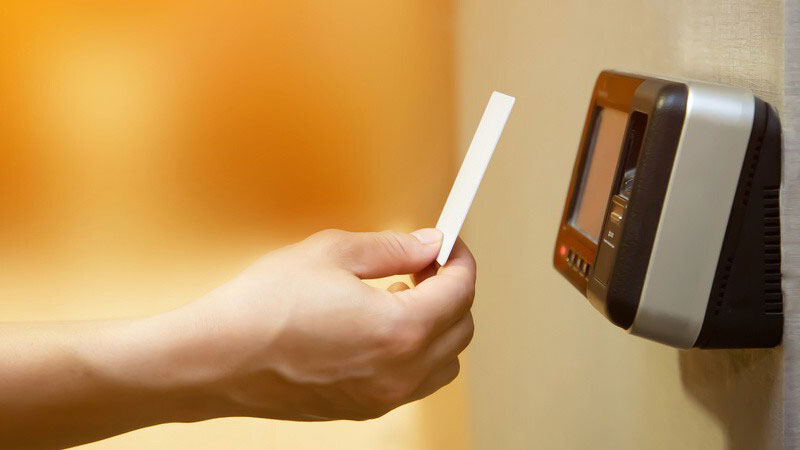The close-up photo captures a white Caucasian male's hand, extending from the left side of the frame, holding a rectangular, white plastic card between the thumb and pointer finger. The card is held just a couple of inches away from a black card reader that features a screen and several buttons beneath it. The background is slightly blurry with an orange-brown hue, and the reader is mounted on a beige wall. The card reader, detailed with a metal strip around its middle, appears to be a keyless entry device, possibly used for secure access in settings such as hotels or other facilities. The white card, devoid of any branding or lettering, is held up for a contactless read by the device.